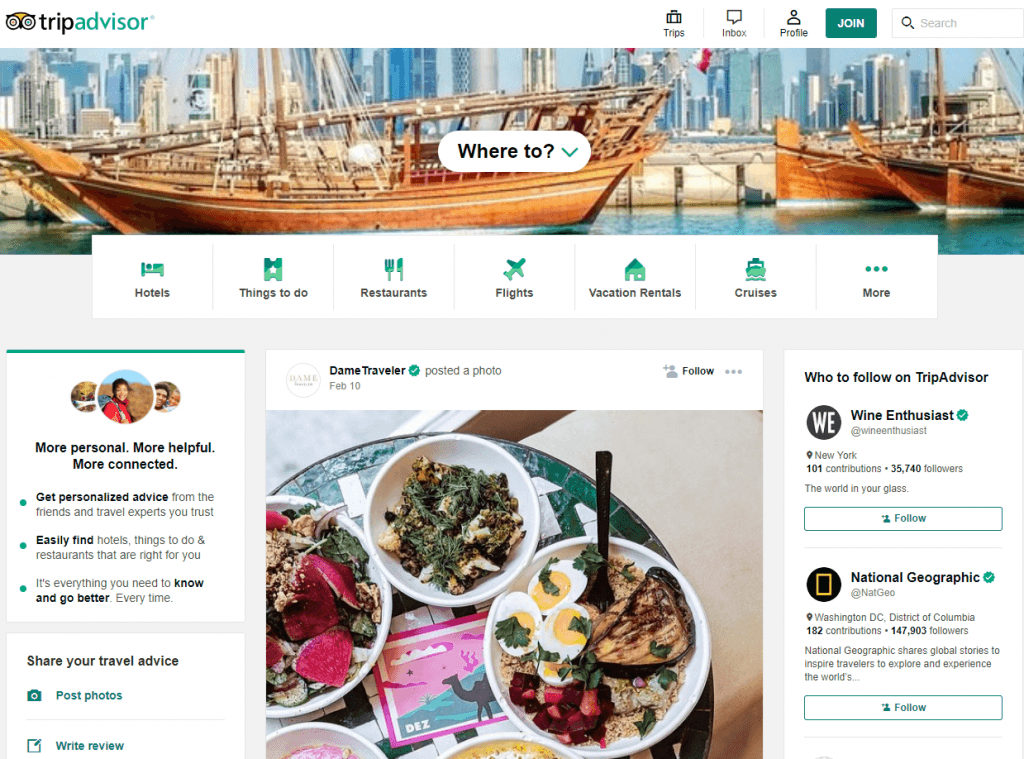### Caption for Image:

This image is a detailed screenshot from a travel-themed website, likely resembling TripAdvisor, featuring various interactive elements and sections. At the top of the page, there are icons for "Trips," "Inbox," "Profile," and a prominently highlighted "Join" button, along with a search box for users to look up travel-related information.

The center of the image displays a banner with illustrations of ships similar to the Santa Maria and La Pinta, set against a big cityscape background. It contains a dropdown menu labeled "Where to?" and options to search for hotels, things to do, restaurants, flights, vacation rentals, cruises, and more through a three-dot menu.

The lower part of the screen is segmented into three primary sections:

1. **Left Section:** This part aims to make users feel more personal, helpful, and connected. It promotes personalized travel advice, easy access to essential information, and encouragement to share one’s travel experiences through photos and reviews.

2. **Middle Section:** Here, a user-submitted photo is showcased. The image features a meal, primarily focusing on a large salad triple serving. A potential postcard on the table hints at the location or context of the dining experience, adding a personal touch to the post.

3. **Right Section:** This segment suggests notable profiles to follow on the platform, including a recommendation to follow National Geographic for enriching travel content.

Overall, the screenshot underscores the website's community-driven approach, inviting users to join a travel blog-like environment where they can exchange advice and share their travel stories.